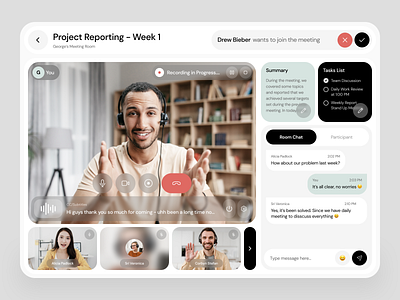This small, horizontal, rectangular image, resembling a slide from a presentation or a Zoom call interface, is encased in a gray border with curved corners. In the upper left corner, the title reads "Project Reporting Week 1." The main focus is a large photograph occupying the left side, featuring a man wearing headphones with a microphone, sitting at a desk, and gesturing with his hands. Behind him, a lamp and bookshelves filled with books are visible, along with drapes. Below this large image are three smaller photographs: one on the left showing a woman in a yellow sweater, the middle one depicting a dog, and the one on the right presenting a man also wearing headphones and a yellow jacket, raising his right hand as if to greet. On the right side of the slide, there is a chat box area with text arranged vertically, summarizing the discussion. The interface overall resembles a Zoom video call, hinting at a collaborative or reporting session.